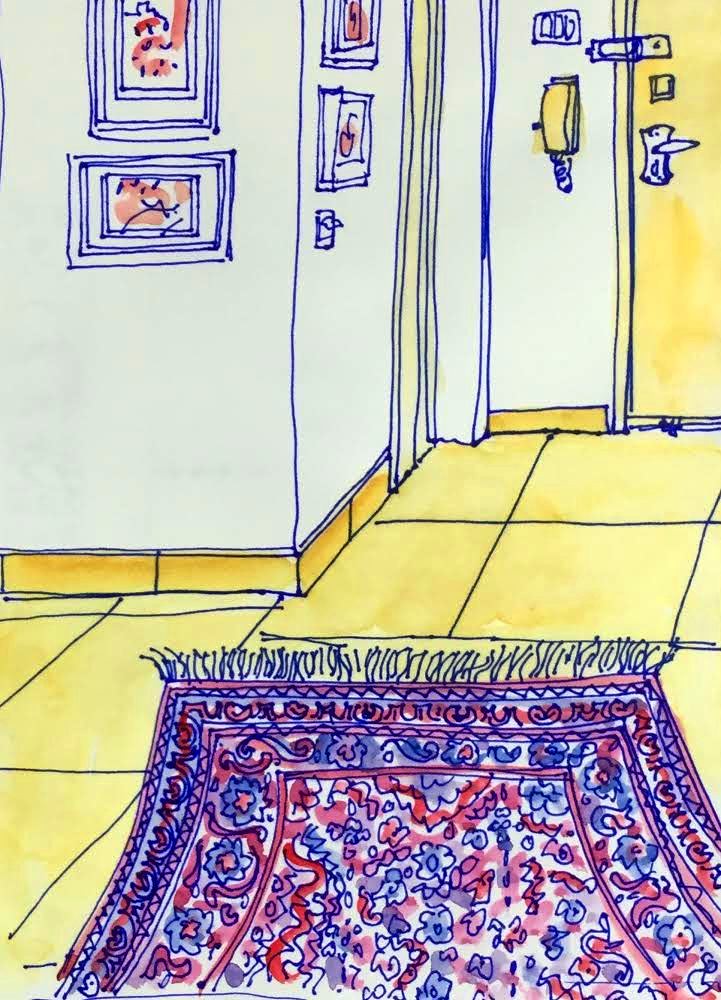The image is a marker-drawn sketch of an indoor scene, possibly an entrance to an apartment, with distinct details. The room has light blue or grayish-white walls with yellow baseboards running along the floor, and a corner where the walls meet. On the right side, there is a yellow door with multiple locks, including a latch and a knob, adding to the sense of security. To the left of the door, mounted on the wall, is an old-style yellow corded phone.

The floor consists of yellow tiles, and near the bottom of the image, a colorful rug with floral patterns in red, purple, and blue stands out prominently. This rug, reminiscent of a Persian design, features frilled tassels at the edges that add texture to the scene. Additionally, the wall displays four framed pictures, providing a sense of lived-in space and personal touch. These detailed elements collectively contribute to the overall atmosphere of a cozy yet somewhat secure entrance.